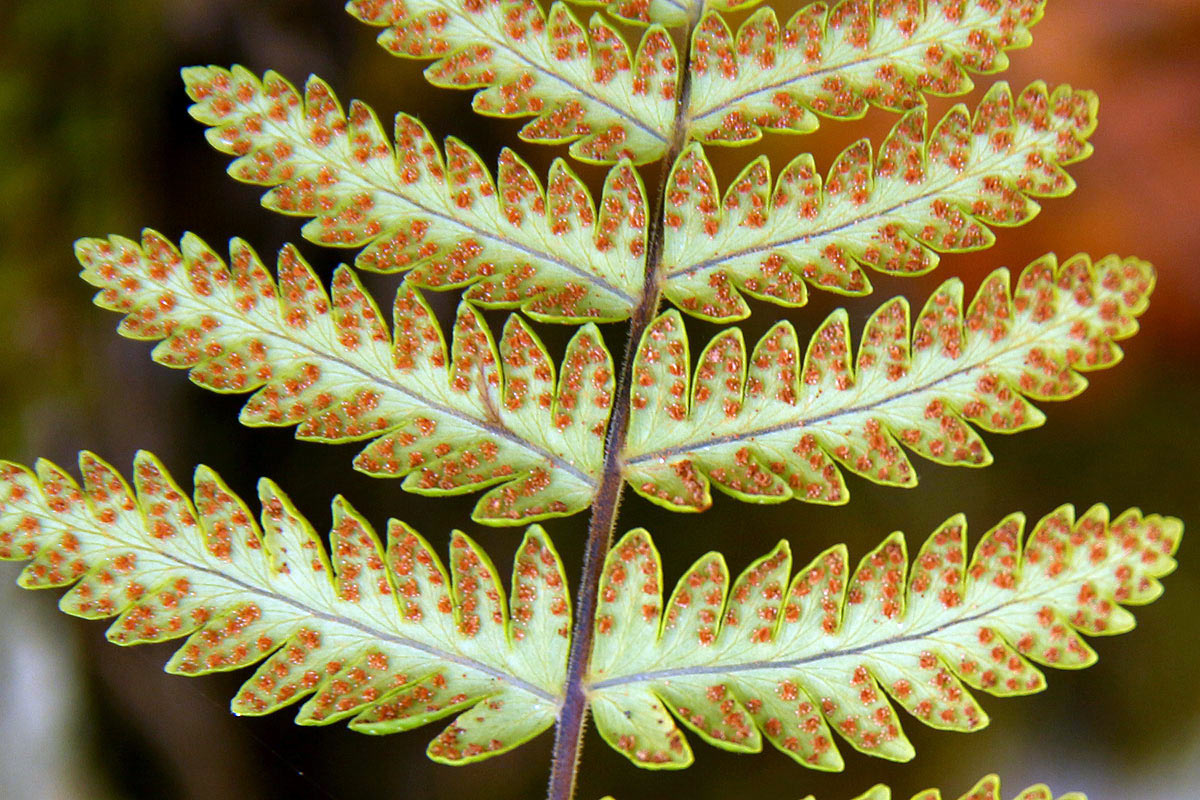This image is a detailed, extreme close-up color photograph of a symmetrical fern leaf, presented in landscape orientation. The fern leaf, which appears to resemble a piece of intricate jewelry, dominates the frame with its stunning, almost surreal beauty. A central stem or twig, brown and slightly slanted to the right, enters the image from the bottom center and extends upward, providing support for the fern's fronds. The fronds, which form a pyramid-like shape, are arranged in four full rows with a fifth partially visible at the top. Each frond is distinguished by a striking pattern: a white center with a dark gray vein running through it, surrounded by a light green perimeter. The edges of the fronds are adorned with orange-red, jewel-like raised areas that add a shimmering texture to the overall composition. The background, blurred to emphasize the fern, exhibits soft green tones at the bottom transitioning to orange hues at the top, suggesting a natural, foliage-rich environment. The photograph showcases a high level of photographic realism, capturing the minutest details of the fern leaf's structure and coloration.